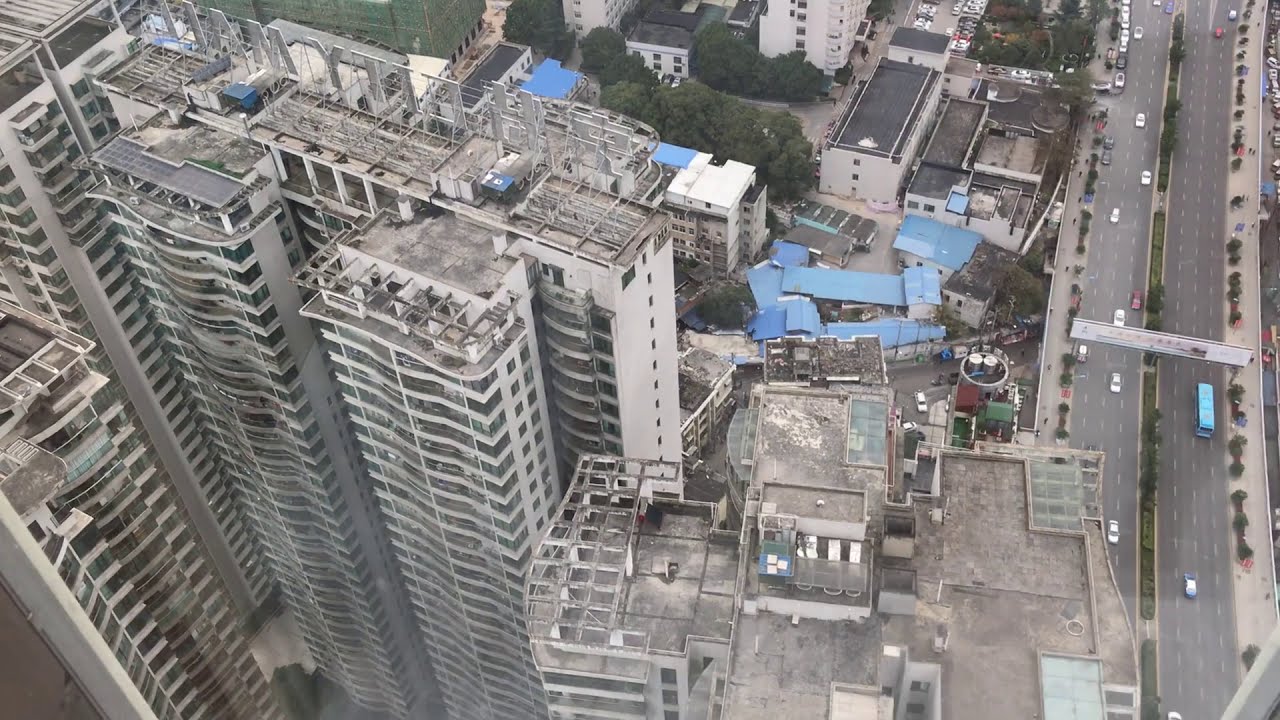This aerial image captures a sprawling urban landscape dominated by towering high-rise buildings, possibly hotels or condos, with numerous balconies. The central high-rise features large signage at its pinnacle, though the text is not visible. To the left of this high-rise, there are smaller white buildings with gray roofs scattered throughout, and a notable blue-roofed structure in the middle of the frame. The right side of the image prominently features a busy eight-lane highway, divided by a green median with trees. This highway also has a pedestrian bridge crossing over it. The presence of a blue bus and numerous cars suggests substantial vehicular activity. The view is likely taken from an airplane or drone, providing a comprehensive top-down perspective that highlights the blend of greenery interspersed among the urban structures. There's also a sign over the highway which might be in Chinese, adding to the city's multicultural landscape.